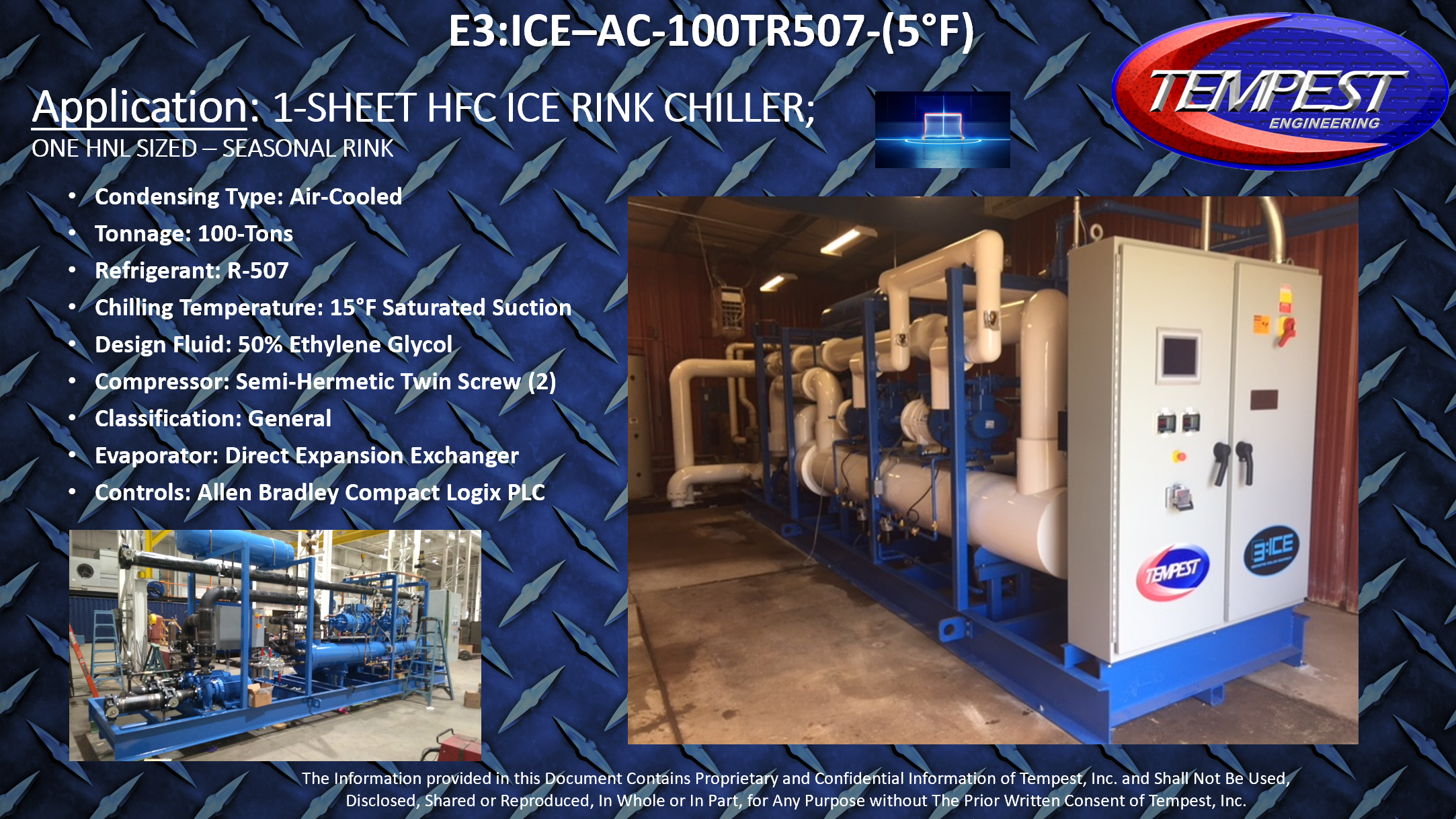The image is a detailed advertisement for Tempest Engineering, showcasing their HFC ice rink chiller. The central text prominently reads "Tempest Engineering Application One Sheet HFC Ice Rink Chiller," describing it as a condensing-type, air-cooled unit with a 100-ton refrigeration capacity using R-507 refrigerant. It has a chilling temperature of 15°F and utilizes 50% ethanol glycol as a drainage fluid. The equipment is visually represented with a machine image located in the bottom right corner, accompanied by another depiction of the warehouse and machinery in the bottom left corner. The color scheme includes blues, dark blues, reds, whites, grays, blacks, and yellows, reflecting a professional and technical aesthetic. The upper right corner features the Tempest Engineering logo in blue and red. The image details its features through nine bullet points and highlights the engineering component’s use in creating ice rinks, suitable for both hockey and ice skating. The overall style of the image is consistent with a PowerPoint presentation or technical advertisement, emphasizing the futuristic design of the ice rink chiller with blue and white piping.